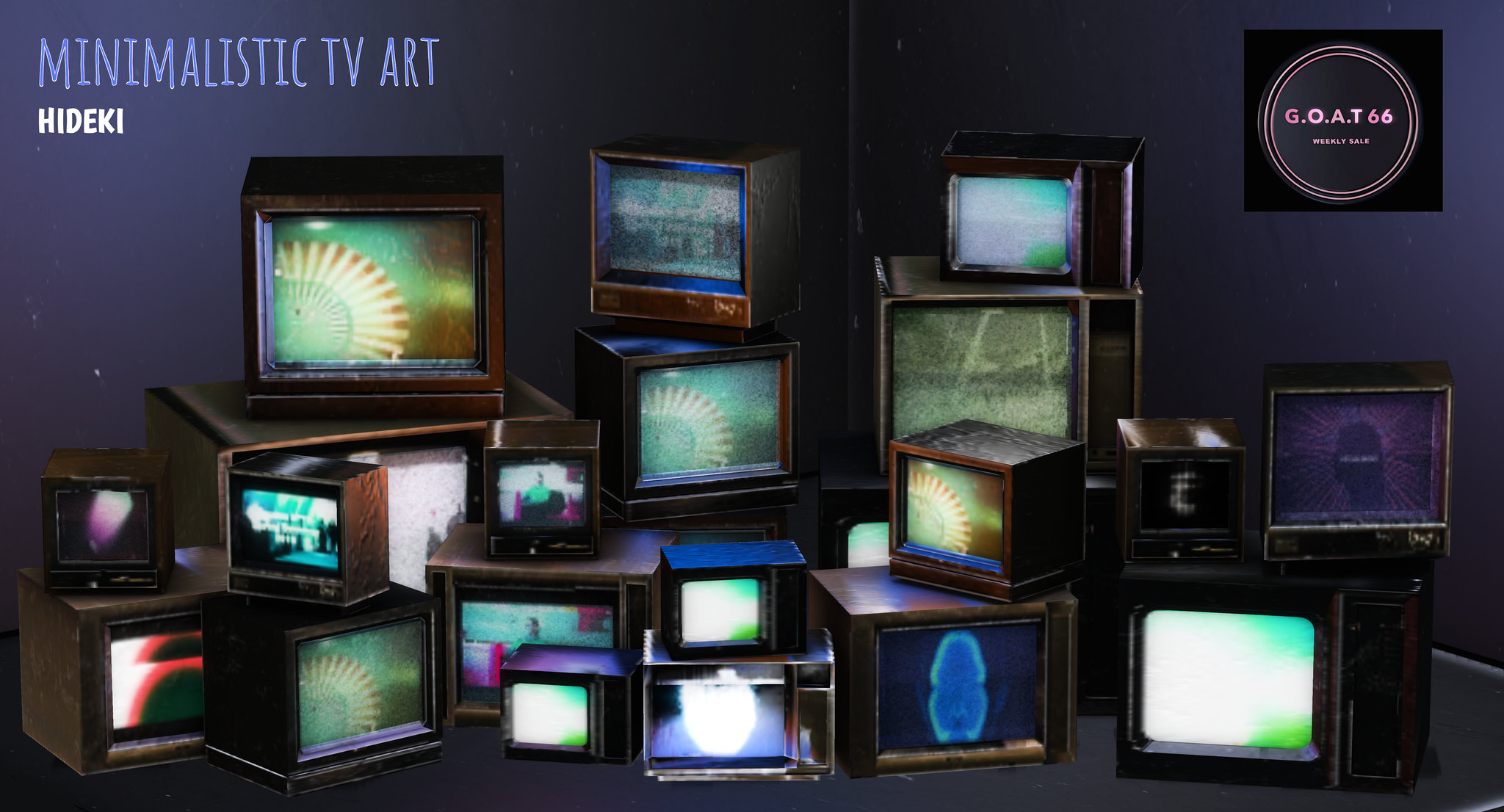The image features a collection of old-fashioned, box-style TV monitors stacked together in a cluttered arrangement, some facing left and others right, resembling a chaotic yet artistic installation. The TVs display grainy, abstract images with dominant hues of green, blue, and occasional bursts of red and pink, lending the composition a vibrant and eclectic aesthetic. Above the TVs, in the upper left corner, bold blue capitalized text reads "Minimalistic TV Art," accompanied by white text underneath that says "Hideki." In contrast, the upper right corner features a black square housing a white circle with the inscription "G-O-A-T 66 Weekly Sale" written inside. The background showcases a room with a solid floor and a dark blue or purple wall, adding depth to the scene and emphasizing the retro-modern theme of the artwork.